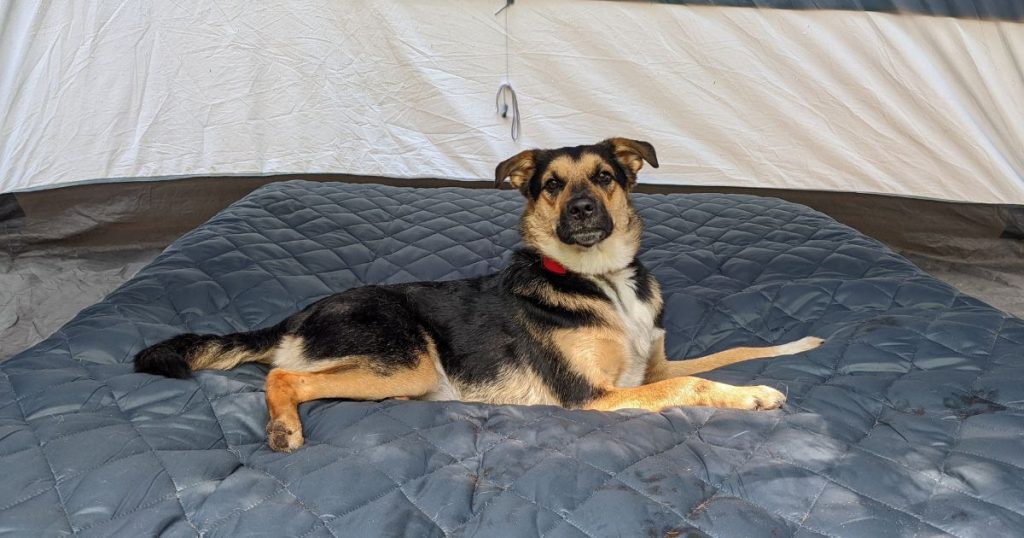The image is a detailed photograph of a dog lying on a blue, diamond-patterned air mattress, situated inside a tent. The dog, resembling a German Shepherd, has a striking coat with black fur on top and brown paws, as well as a brown face with black fur around the eyes and nose. The dog is positioned at the center of the mattress, lying still with eyes wide open, staring directly at the camera. Long drooping ears and a long tail are visible. The background reveals the white walls of a tent that stretch from left to right, with a rope or string hanging down from the top center. The bottom of the tent has a black strip and gray material, with hints of grass peeking from the left and right sides. The floor beneath the mattress appears to be brown, contrasting slightly with the tent's light gray bottom material.